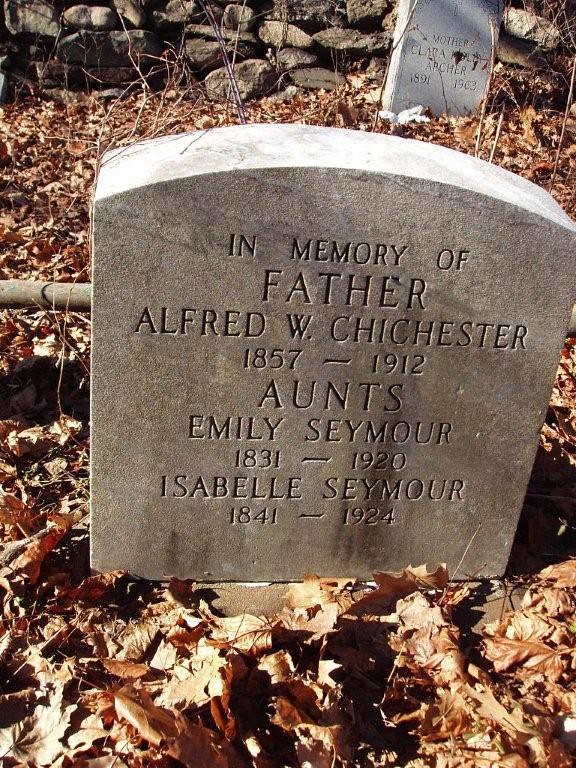In this tall rectangular color photograph taken outdoors on a sunny day, a granite tombstone stands prominently on a surface covered in dried brown leaves, suggesting it is autumn. The tombstone, situated slightly left of center, is engraved in all capital letters with the inscription: "In Memory of Father Alfred W. Chichester, 1857-1912. Aunts Emily Seymour, 1831-1920. Isabelle Seymour, 1841-1924." To the right in the background, there is another tombstone, smaller in size and slightly curved at the top, which reads "Mother Clara Archer, 1891-1963." Behind these tombstones, a brick wall made up of irregularly shaped gray stones can be seen, along with a horizontal post or pipe on the left side of the primary gravestone. The photograph's lighting comes from the upper left, highlighting the textured surfaces and the tranquil, somber atmosphere of the gravesite.